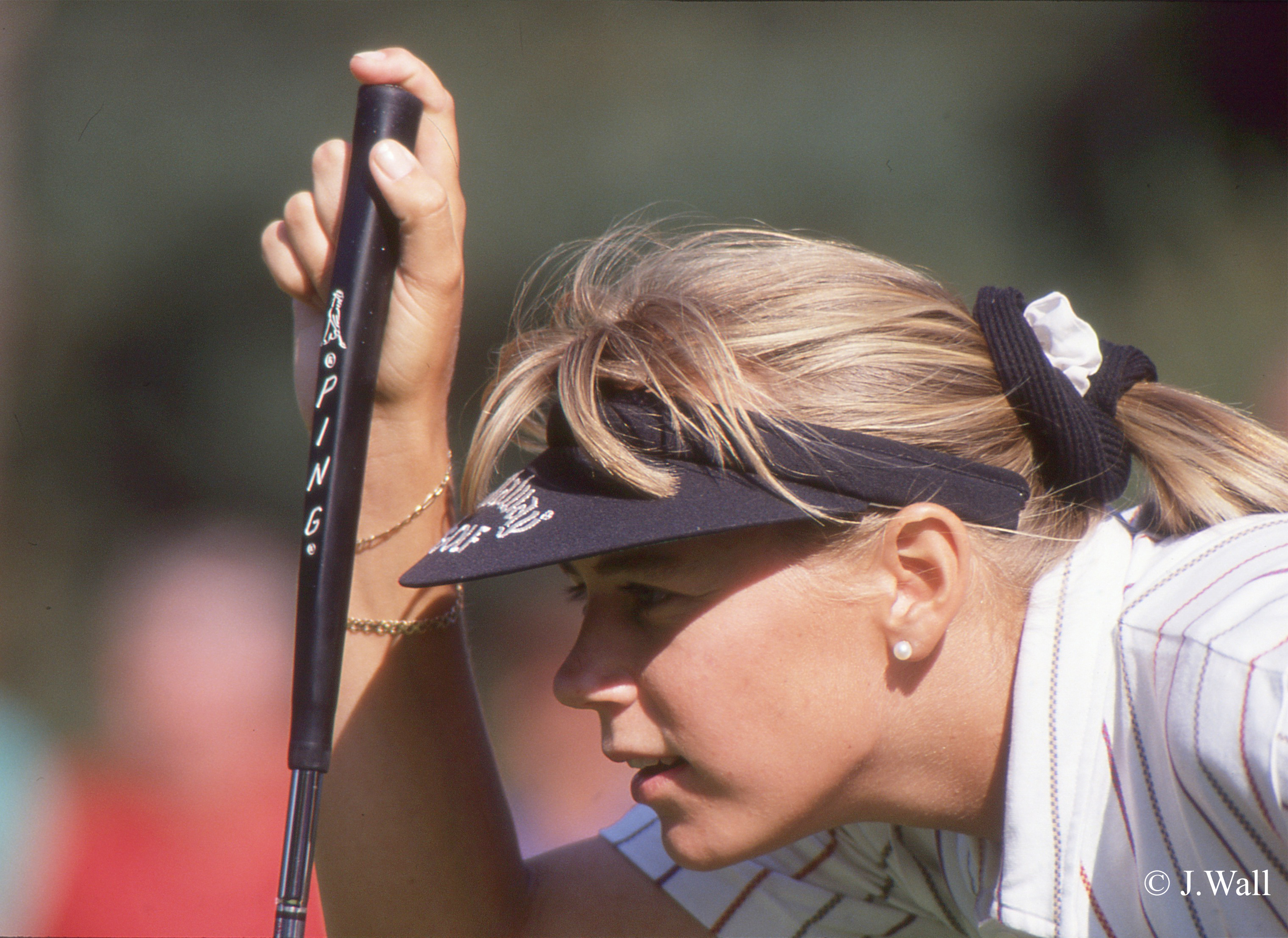The photograph captures a woman in her late 20s or early 30s, focused on her golf game. Sporting long blonde hair pulled back into a ponytail with a black and white scrunchie, she kneels down, intently gazing at an unseen object off-camera, likely the golf ball or the field. She wears a black visor with white Callaway Golf lettering to keep her bangs off her face, and her ears are adorned with simple pearl stud earrings. Her right hand firmly grips the black handle of a Ping golf club, inscribed with the word "PING" in white. She wears a white polo shirt, patterned with multiple red zigzag stripes, and her wrist is embellished with two gold chain bracelets. The background is blurred, hinting at a grassy area with indistinct figures, and the bottom right corner features a white watermark reading "copyright J. Wall."